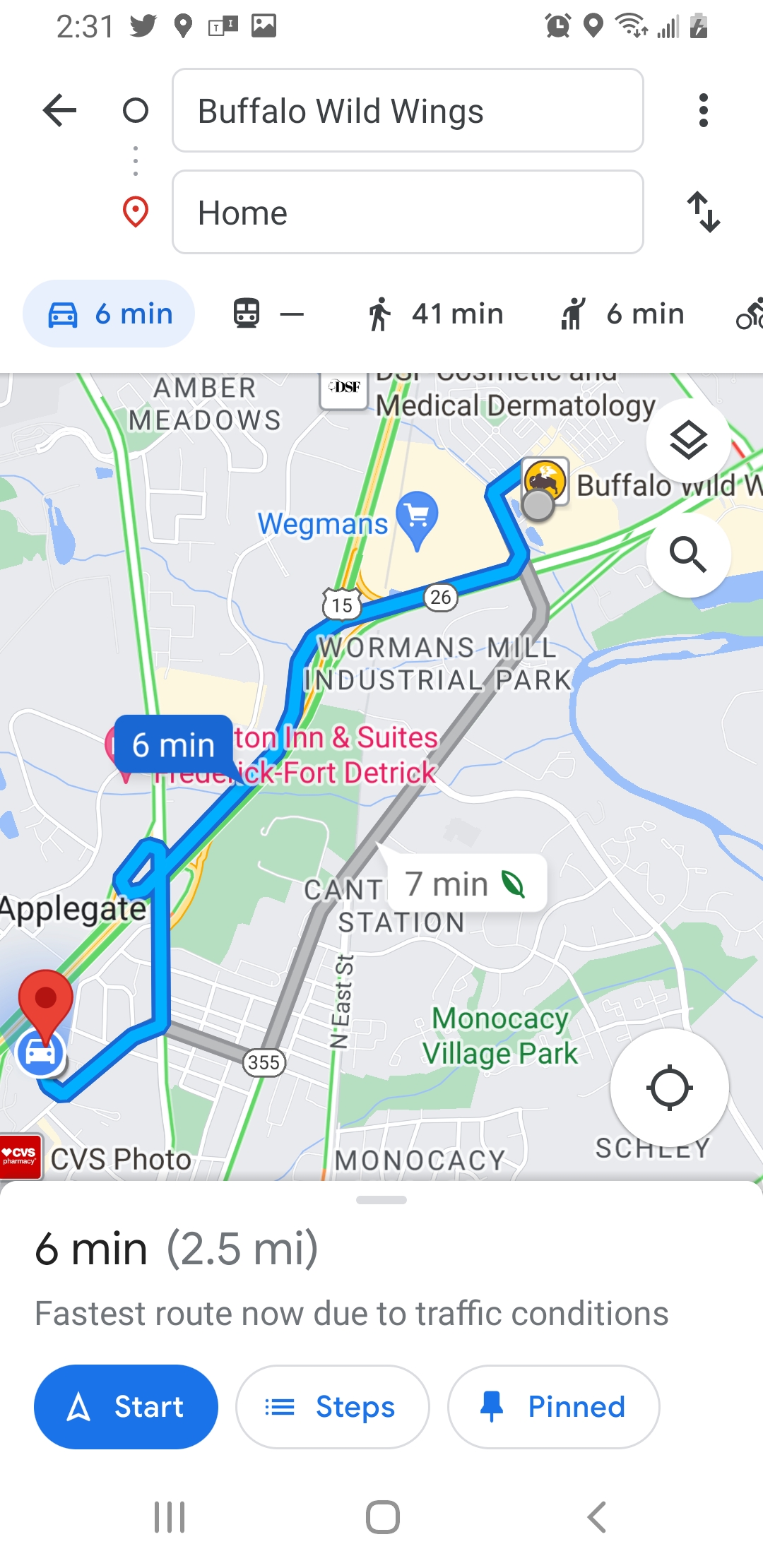This screenshot from a phone displays a Google Maps interface detailing a route from home to Buffalo Wild Wings. The top left corner shows the number 231, flanked by Twitter icons on either side. The status bar on the right indicates an alarm clock, Wi-Fi connection, signal strength, and battery life. Below the status bar is a search bar with "Buffalo Wild Wings" entered, and a location pin icon representing the current position labeled "home." The map showcases a route with blue-highlighted streets for the main path, alongside green and gray streets. Locations along the route include Monocacy, Applegate, Amber Meadows, Warman's Mill Industrial Park, Norman's Mill Industrial Park, Hampton Inn and Suites, Fort Detrick, and Monocacy Village Park. The map indicates a 2.5-mile distance, taking approximately 6 minutes by car, with alternatives for public transit, walking (41 minutes), and other travel modes. The fastest route is tagged due to current traffic conditions. At the bottom are three buttons: a blue "Start" button, a white "Steps" button with blue lettering, and another white button labeled "Pinned" in blue.